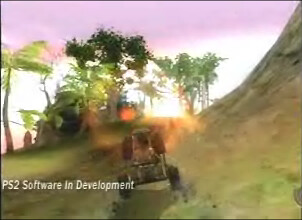The image is a small square snapshot featuring a scene from a video game. In white text at the bottom, it reads "PS2 Software and Development." The scene showcases a go-kart, or a similar small vehicle, captured from behind as it emits flames from its front. The setting is a vibrant jungle with towering palm trees dominating the left and center background, while a large hill rises on the right. The ground beneath the cart is a lush green, and the sky above transitions from a deep purple at the top to a fading white toward the horizon. A prominent sun glare occupies the center of the image, suggesting bright sunlight reflecting off the camera lens.